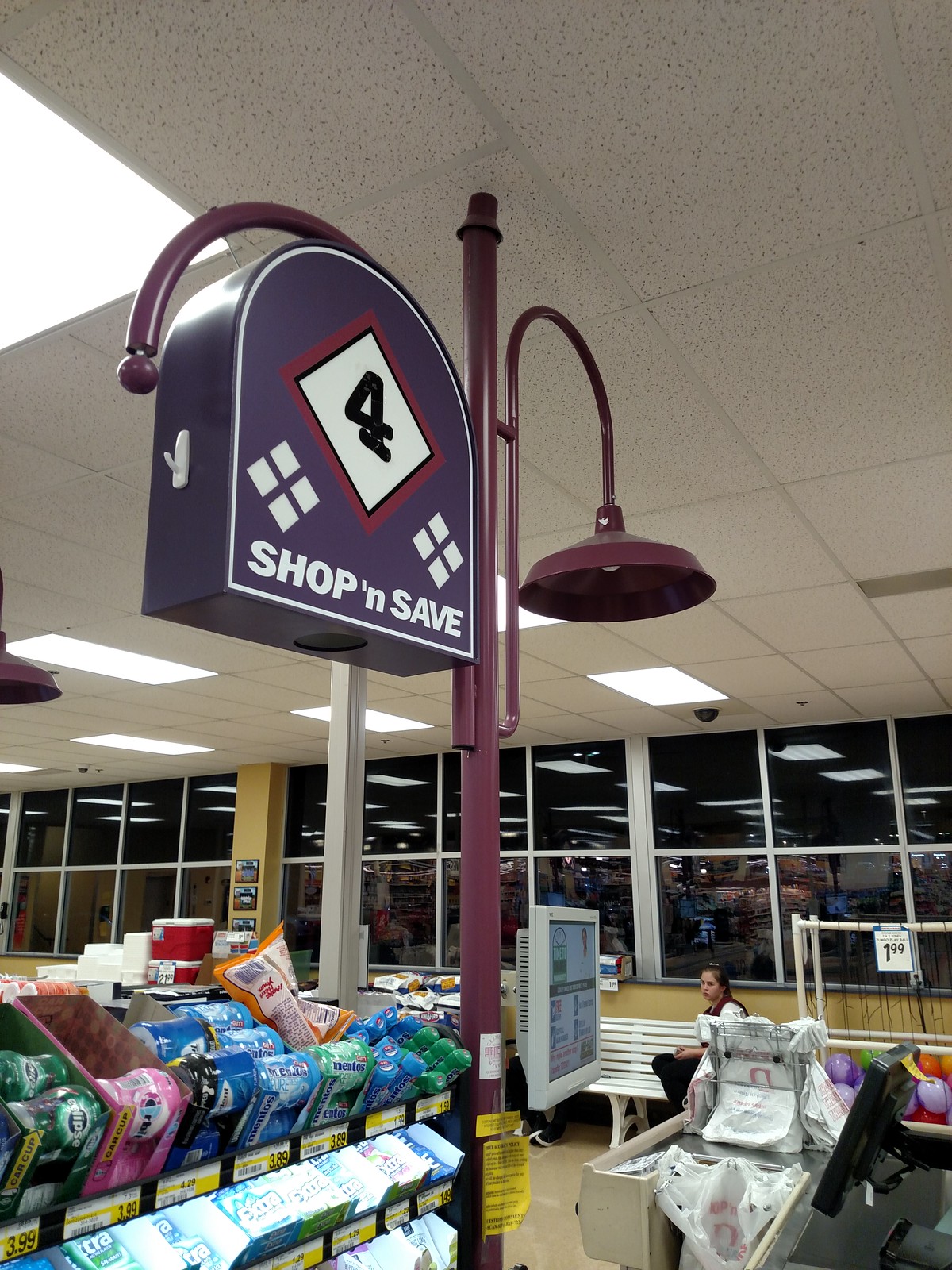Inside the grocery store, a striking scene unfolds featuring a metal pole at the center. This pole branches out in two directions: one arm rises up, bends downward, and supports a brown lamp fixture, while the other arm curves downwards, terminating in a "Shop and Save" sign marked with the number four. Hanging from the side of this sign is a small plastic hook.

The store's back wall, behind this central installation, is lined with large windows, allowing natural light to flood the space. Below these windows, a long white bench stretches across the area. A girl, dressed in a white shirt and black pants, is seated on this bench.

Next to her, there's an intriguing setup: a small pit constructed from PVC pipes and netting, filled with colorful balls priced at $1.99 each. Moving to the left of the bench, there's a prominent display of Kingsford charcoal bags. Further left, the scene transitions into a candy aisle, teeming with assorted sweets.